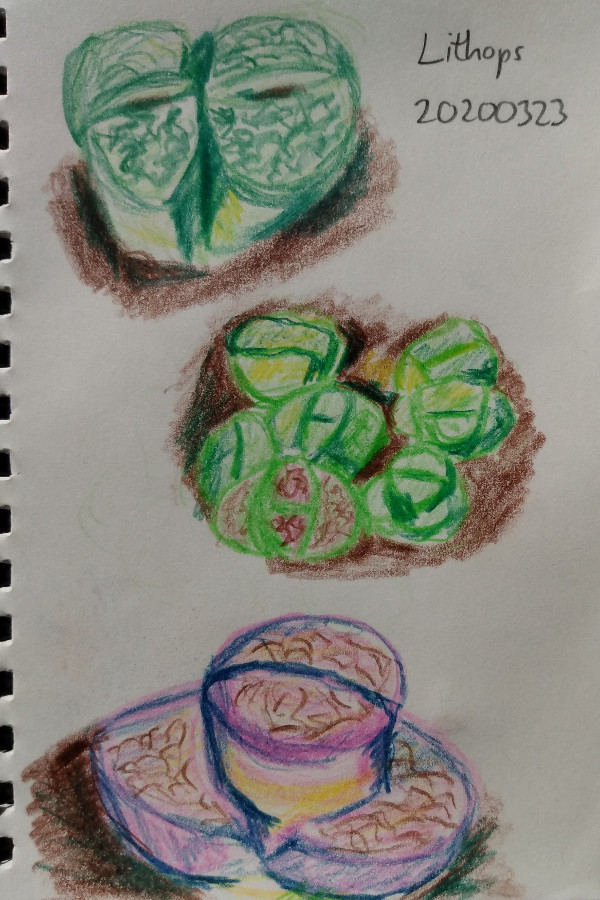This image features a detailed sketch on a light gray notepad. In the top right corner, the word "LITHOPS" is inscribed in bold black text. Below it, the code "T-2020-0323" is also written in black. The left side of the notepad includes a vertical dotted line running along the edge. 

At the bottom of the page, there is a detailed drawing comprised of several objects. The lowest object is a flat, circular shape, topped by a drum-like structure, all rendered in shades of brown, pink, yellow, and blue. Above this, there is a brown-shaded area filled with numerous green circles. To the left of this section, another brown-shaded area contains two green objects situated in its upper-left corner.